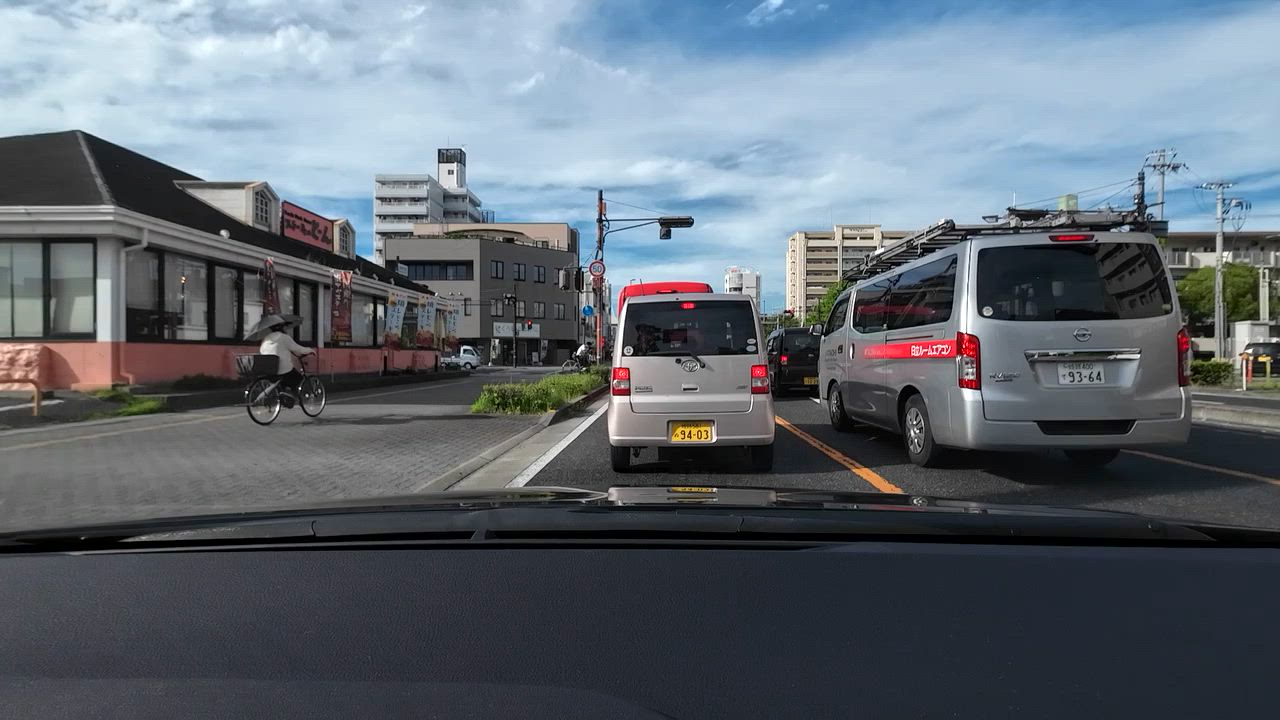This photograph captures a bustling street scene in Canada. Taken from inside a vehicle looking out through the windshield, the image shows a line of vehicles, including several vans and a car, moving along a blacktop road. On the left side of the frame, a bicyclist is approaching a crosswalk, seemingly about to cross in front of the vehicles. The sky above is a clear blue, adorned with wispy white clouds, adding a serene backdrop to the busy urban environment. On the left side of the street, a row of buildings housing businesses and hotels can be seen, contributing to the city's commercial atmosphere. The right side of the street features a mix of power lines, trees, parking lots, and additional buildings, framing the scene with a typical urban landscape.